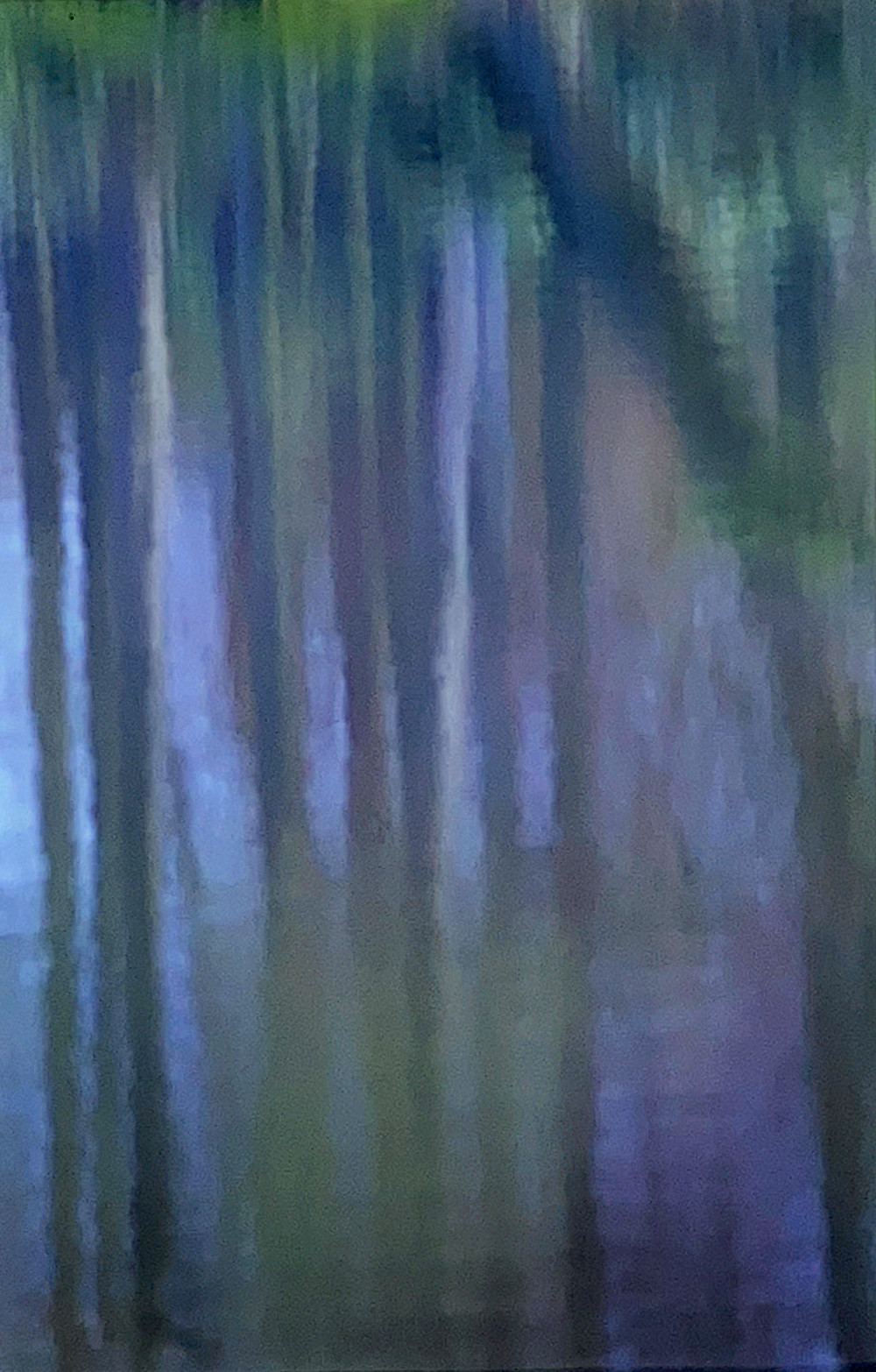The image is an abstract painting characterized by a blurred, indistinct quality. It predominantly features a mixture of vibrant colors that blend together in a smearing pattern. Starting at the bottom left, the colors transition from brown, beige, and caramel light brown to yellow and various shades of green. As you move towards the center, these colors intermingle, with green and blue smears becoming prominent, alongside patches of white, maroon, and darker gray. On the right-hand side, there is a mix of purple, periwinkle, and dark green hues, which continue to blend towards the center.

Descending smears, particularly of green, blue, and white, dominate the composition, with intermittent maroon and gray streaks. There are notable green smears at the top, accompanied by white and blue at the bottom. One distinct feature is a smear that moves dynamically from the bottom right corner upwards, swooping leftward, combining black on the top and brown on the bottom.

Additionally, the blurred strokes and unevenly spaced, descending green streaks give an impression of natural elements, possibly evoking the form of a tree or branches hanging over water. The midnight blue background further amplifies this effect, mingling with hints of imagery that could resemble a boat and water, suggesting a serene, watery landscape hidden within the abstract blend of colors.